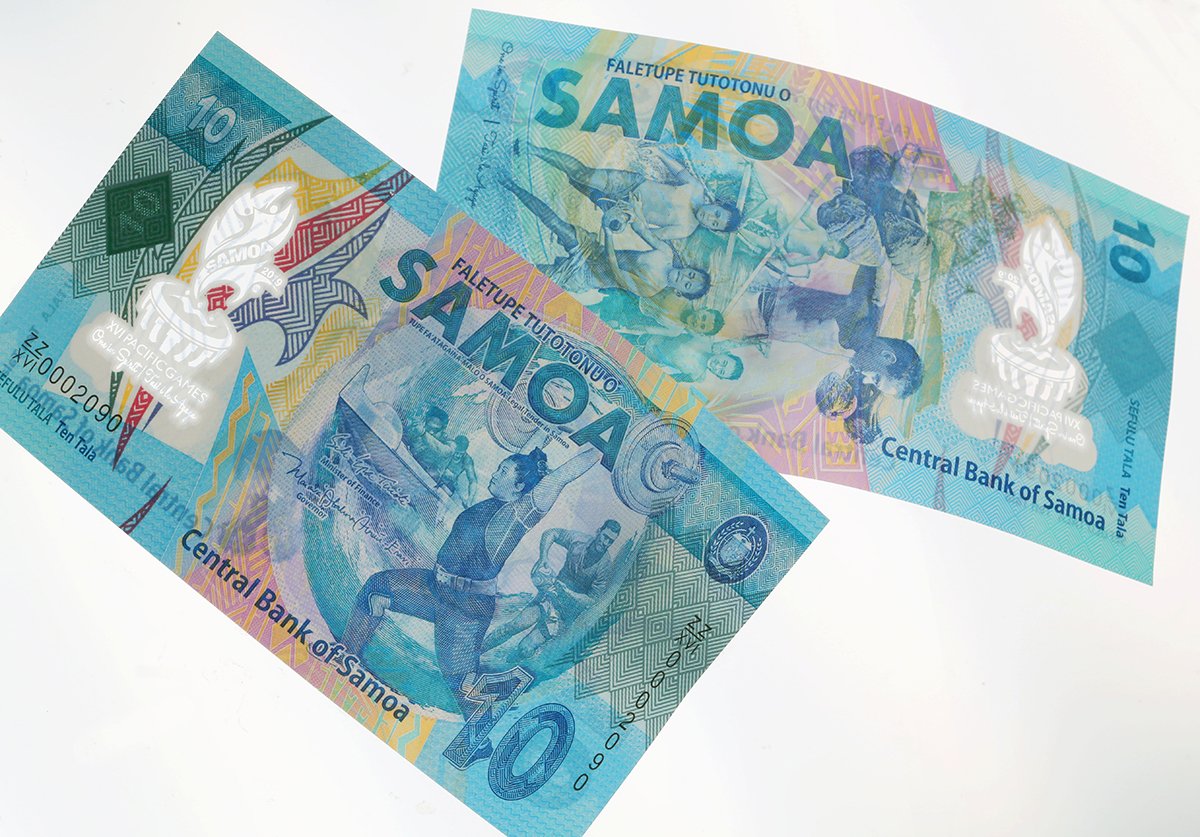This detailed photograph displays both the front and back sides of a ten-unit bill from the Central Bank of Samoa. Each side prominently features the text "Falatupu Tutonu," and "Samoa." The primarily light blue bills also incorporate shades of yellow, red, and navy blue in their intricate design. 

On the front side of the bill, a weightlifter dressed in a short-sleeved jumpsuit and tennis shoes is depicted. The background includes swirling wave patterns and the country name "Samoa" set against a white flame-shaped symbol. 

The back side of the bill illustrates athletes engaged in various activities, possibly playing a ball game or boxing, suggesting the prowess and cultural importance of sports. One athlete is depicted carrying a stick with fruits, possibly coconuts, emphasizing the native elements of the island. Both sides of the bill show a serial number, although only one can be seen clearly in the image.

Overall, the detailed imagery and vibrant colors reflect the cultural and athletic heritage of Samoa, embedded within the ten-unit currency notes.